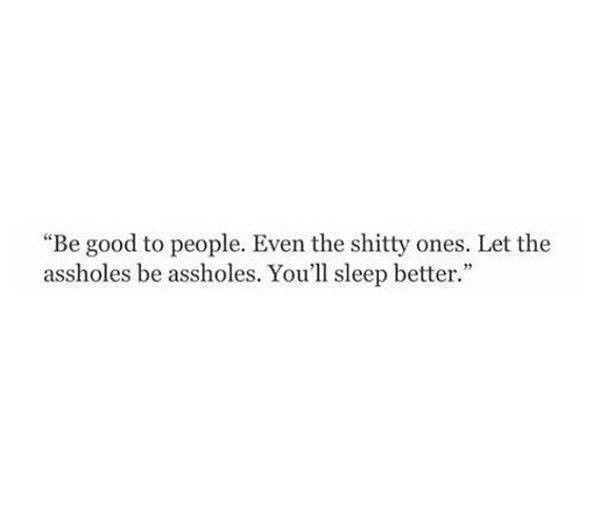The image is a square with a plain, white background that is completely empty and uninteresting. The focal point of the image is a centered, inspirational quote rendered in a font resembling Times New Roman. The black text is presented in two lines, using proper capitalization, and reads: 
"Be good to people, even the shitty ones. Let the assholes be assholes. You'll sleep better."
Behind the text, there is a subtle, grainy texture that adds a bit of depth to the otherwise stark background. The text stands out clearly due to its contrast against the white background, making the message the central and sole focus of the image.